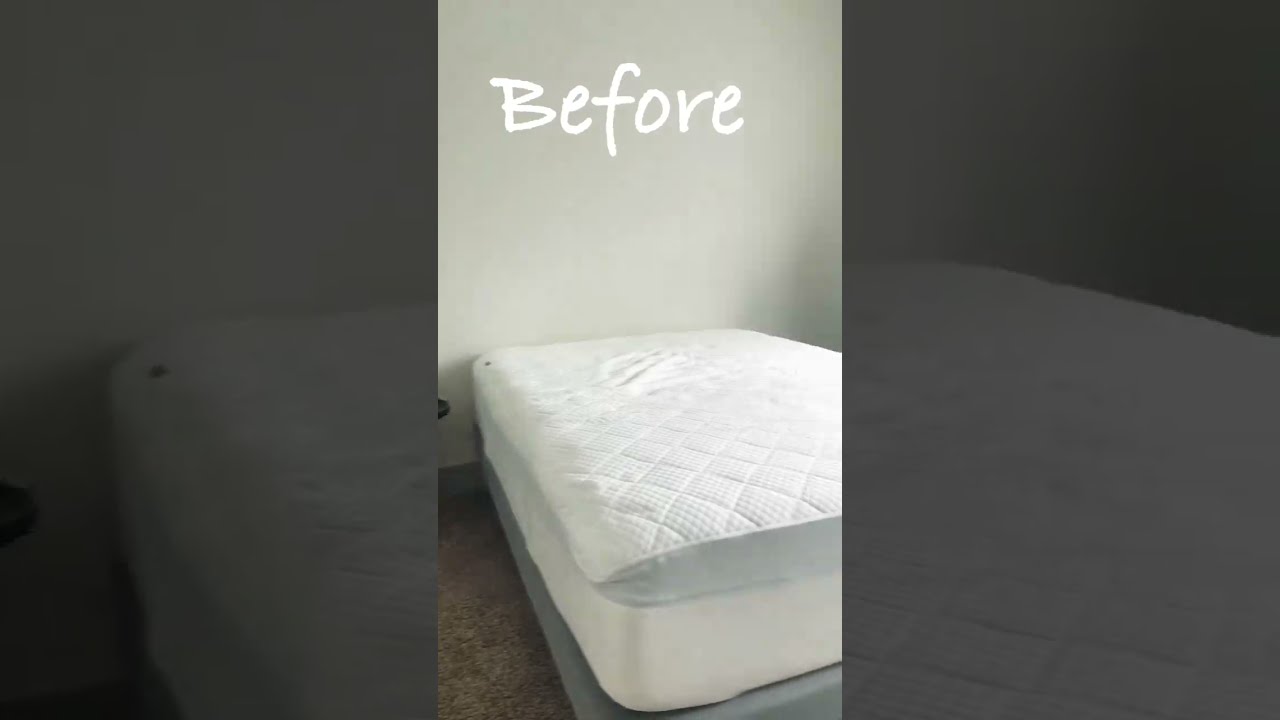In a sparse, white-walled room, a thick, white mattress with a diagonal, diamond-patterned topper lies atop a gray box spring, all perched on a brown carpet. The mattress shows slight signs of wear but remains clean. Shadows stretch along the right side of the wall, emphasizing the vertical shot, likely captured from a cell phone, possibly for a video or social media post. Above the scene, white text reads "Before." The image is duplicated in the background, larger and darker, creating a backdrop effect. A hint of an outlet can be seen on the left side of the wall. The overall color palette includes white, gray, black, brown, tan, and silver, contributing to the minimalist aesthetic.